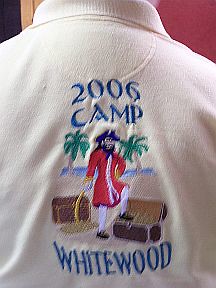This close-up photo captures the back of a person wearing a white pullover shirt with a collar. The focus is on the detailed design on the shirt, which reads "2006 Camp Whitewood." The graphic features a pirate dressed in a vibrant red outfit, with a black beard and a black hat. The pirate brandishes a sword in his right hand while his left hand rests confidently on his hip. His left foot is propped up on an open treasure chest, revealing gold and treasures. A second closed treasure chest is situated behind him. The background showcases an ocean scene with two swaying palm trees, adding to the adventurous atmosphere of the pirate-themed image.